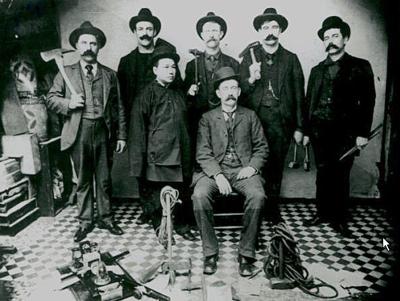This rectangular black and white photograph, taken indoors, captures a group of seven men positioned against a white wall. The back row features five standing men, all Caucasian, adorned in old-fashioned suits, wide-brimmed hats, and sporting prominent mustaches. Each of these men holds various tools reminiscent of laborers or workers, including axes, hammers, and possibly steel posts. In front of them, on a floor tiled in a black and white checkerboard pattern, stands a younger boy and a shorter gentleman. Next to the boy, a man sits in a chair; he appears Asian among otherwise white individuals. The floor is cluttered with cords, ropes, and pieces of equipment, while off to the side, a statue resembling a dog and other objects, potentially boxes or stairs, add depth to the scene. The meticulous arrangement of the men and their tools suggests they are poised for a formal yet industrious group portrait.